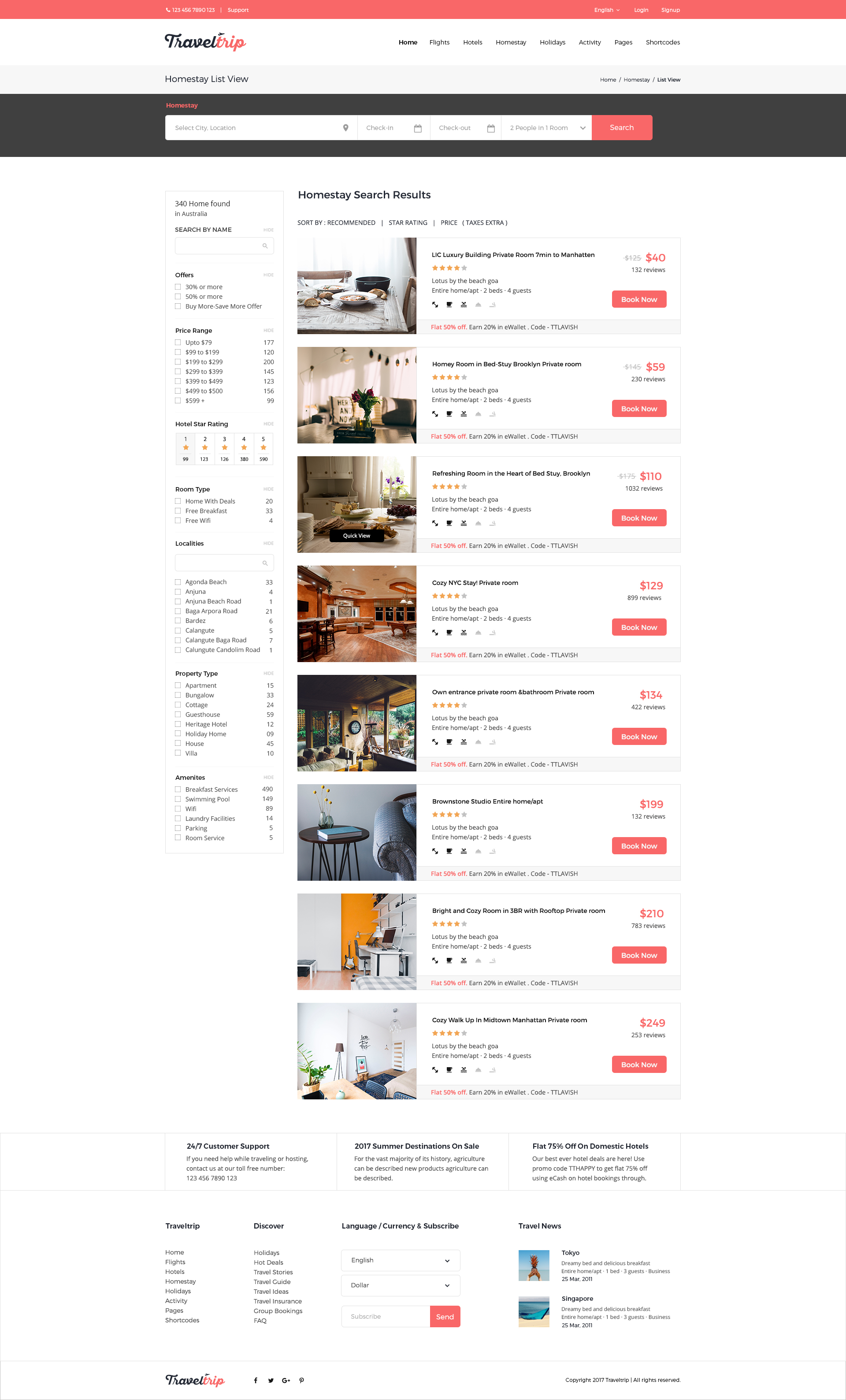The image is a screenshot from a mobile phone display showing an online homestay booking website, likely named "Homestay Last" or "Homestay List View." The webpage is titled "Homestay Search Results." At the top, there are options to "Sort By" recommended items, star rating, or price. The header also includes filters for "Select City and Location," "Check-in," and "Check-out" dates, with options for "2 people in 1 room." A prominent search button in a reddish-orange hue is visible.

The left sidebar indicates there are "340 homes found" in Australia. Users can search homes by names or select from various offers like "30% or more," "50% or more," or "Buy More, Save More." The price range filter spans from "$79" to "$599+."

Additional filters include host star ratings from one to five stars, room types, deals offering free breakfast or free Wi-Fi, and locality details such as nearby beaches. Property types and available amenities are also listed.

The main body of the screen features a scrolling gallery of images showcasing various homes available for booking.